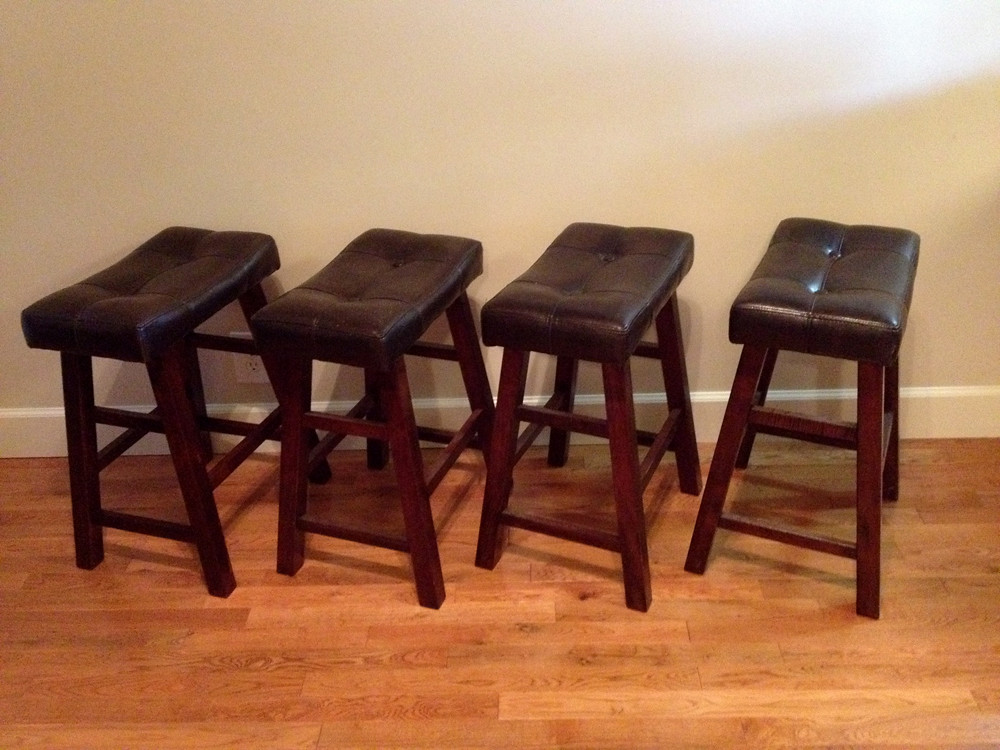The image captures four identical barstools arranged neatly against a cream or beige-colored wall with a white baseboard trim. Each stool showcases dark cherry wood legs paired with a rectangular, plush brown leather seat cushion, suggesting a comfortable seating experience. The stools are uniformly aligned on a nicely polished hardwood floor. By the leftmost stool, the wall features a visible white electrical outlet. The setting appears to be a home environment, possibly indicating the stools are either part of a new interior setup or positioned for sale on platforms like Facebook Marketplace or Kijiji.